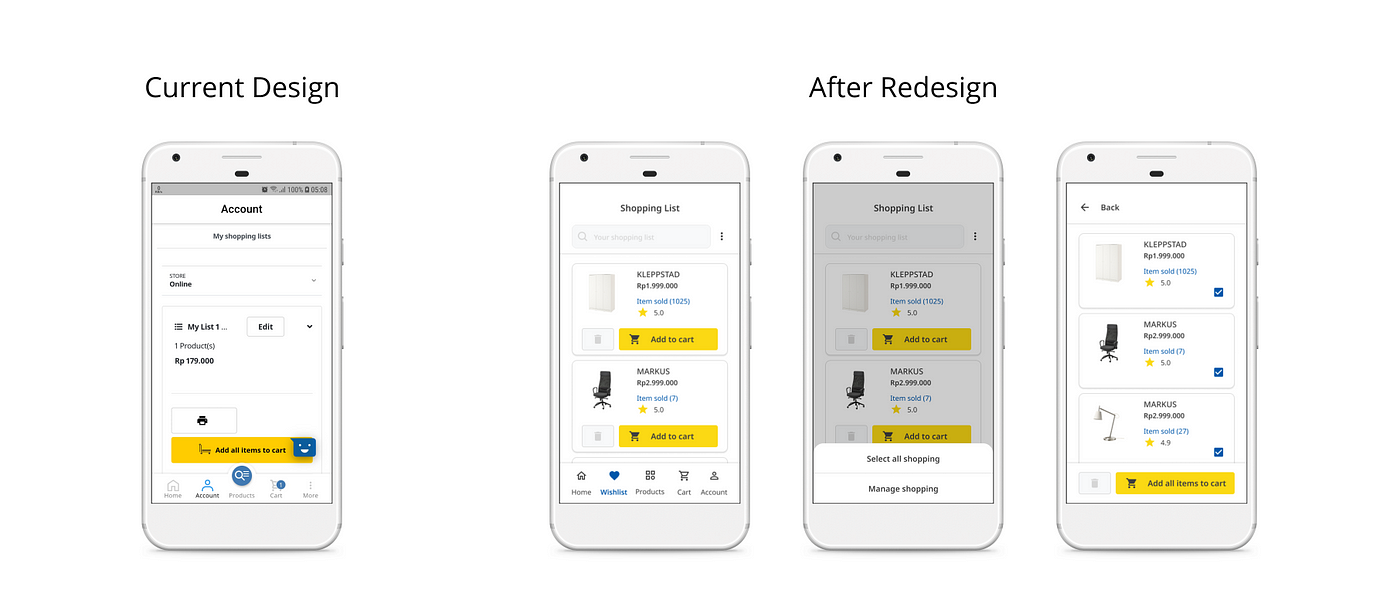This screenshot showcases four mobile phones displaying different app interfaces. The first phone on the left illustrates the current design, characterized by a sleek white exterior and a matching white interface. Contrasting elements such as the word "Account," boxes, and arrows are rendered in black for clear visibility. The screen prominently features the word "Account" along with three chair icons representing different versions of a shopping list interface, as opposed to a singular "My List" option. Notably, the interface integrates yellow buttons, adding a splash of color to the otherwise monochrome scheme.